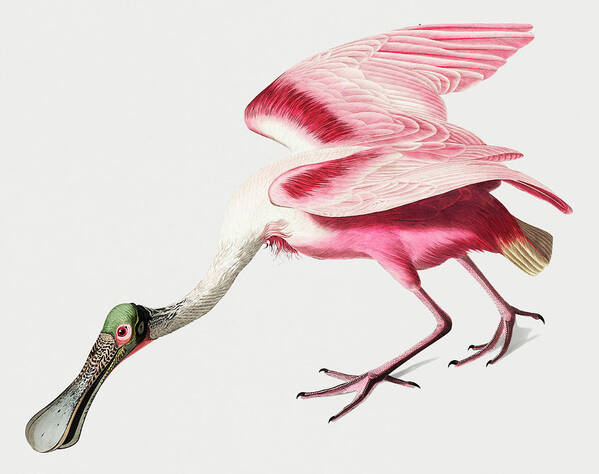This image showcases a vibrant depiction of a Rosé Spoonbill in a square, borderless print against a light gray background. The bird, striking in its multi-colored feathers, features a predominantly pink body with darker patches on the upper wings and pristine white tail feathers. Its long, slender white neck arches gracefully downward, giving the impression that the bird is poised to hunt or forage. The Spoonbill's small green head boasts a distinctive long, flat, black bill, resembling a spoon, and underlining its unique characteristics. Notably, the left eye is highlighted with a white circle, accented by a touch of pink beneath it. The bird stands with its left foot slightly ahead of the right on an otherwise minimalistic white surface, casting subtle shadows. This artistic piece captures the essence of the Rosé Spoonbill's elegance and distinctiveness, emphasizing its captivating coloration and form.